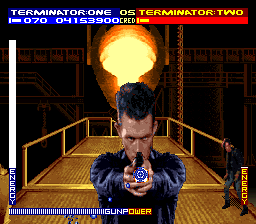The image appears to be a screenshot from an older video game. It portrays a small square frame with several distinct elements. At the top of the frame, there is the text "Terminator 1070-04153900" with a blue background, and next to it, the title "Terminator 2" stands out on a red background with yellow writing. The scene within the frame shows an explosion in the backdrop, flanked by rudimentary-looking stairs and a walkway.

In the foreground, a male character is central to the action. He is depicted facing the camera, holding a gun with both hands extended as if he is about to fire. On the lower right side of the image, another smaller figure is visible. This character is less detailed and is dressed in a black shirt, blue jeans, and black shoes. 

Additional text elements are embedded within the image: the word "Energy" is written vertically next to the smaller figure in small print. Along the bottom of the frame, "Gunpower" is displayed, and to the left side, "Energy" appears with blue lettering on a blue background. Blue lines scatter across the frame, contributing to the graphical style characteristic of vintage video games.